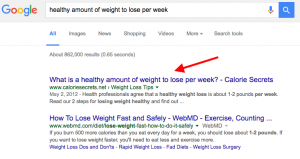A screenshot of a Google search results page depicts several online resources addressing weight loss. At the top of the page, the word "Google" is prominently displayed, followed by a search bar containing the query "healthy amount of weight to lose per week" inside a gray box. Beside the search bar, there are microphone and blue square search icons. Below this, a menu bar offers options such as "All," "Images," "News," "Shopping," "Videos," and "More."

The search yields approximately 882,000 results. The first search result is highlighted by a large red arrow pointing to the phrase "weight to lose," leading to a website named "Calorie Secrets" (www.caloriesecrets.net), which offers various weight loss tips. The second search result is from WebMD, titled "How to Lose Weight Fast and Safely." This link suggests practical methods for weight loss, such as burning 500 to 600 more calories per day to achieve a loss of one to three pounds per week. The screenshot ends here, summarizing only these top two results.